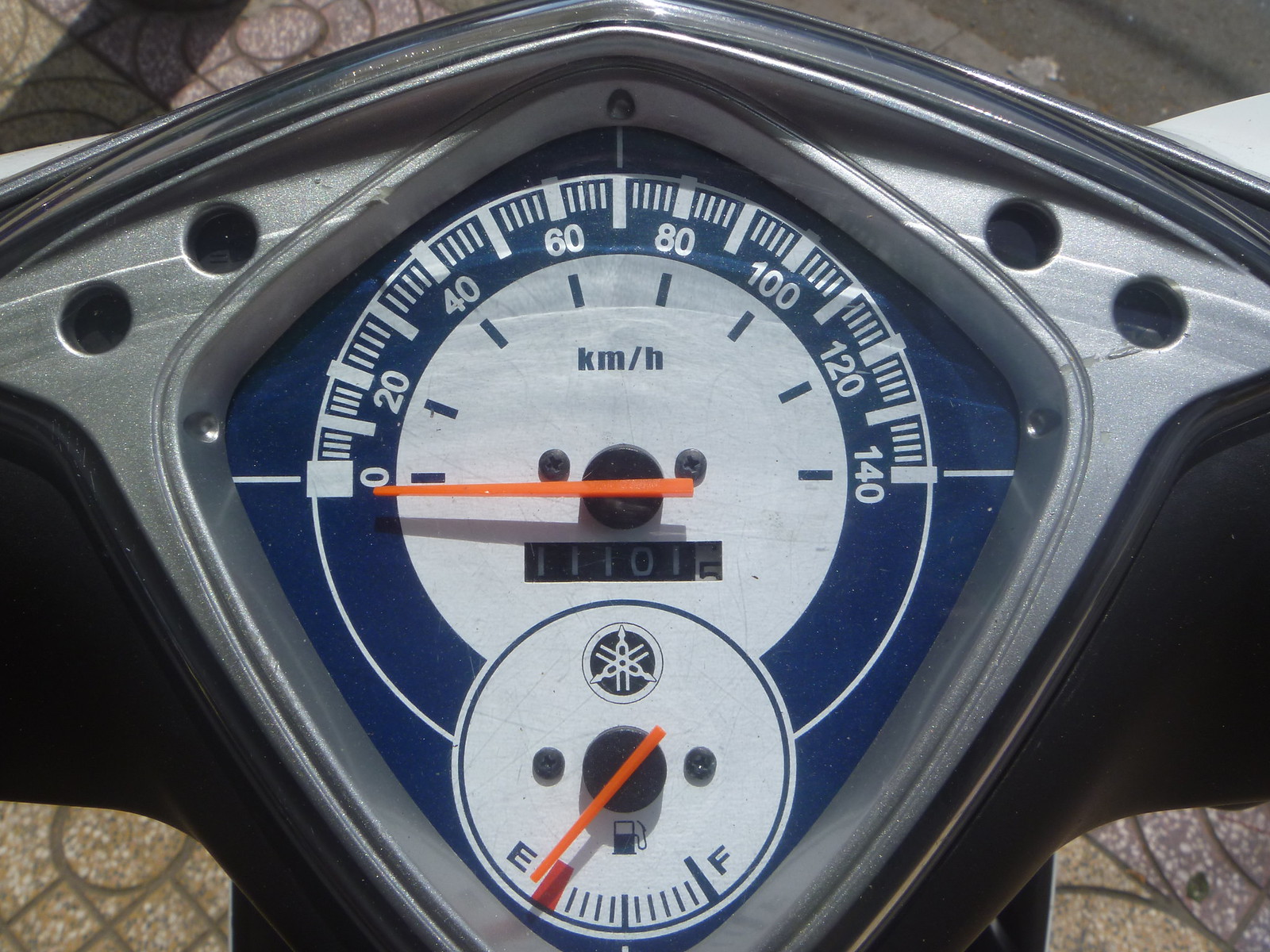This photograph captures a first-person, top-down view of a motorcycle gauge cluster, prominently showcasing a classic analog speedometer. Encased in a sleek, stainless steel bezel, the central speedometer features a blue background with a clearly marked scale reading up to 140 kilometers per hour. The vibrant orange needle rests at zero kilometers per hour, indicating that the motorcycle is stationary. Below the speedometer, the odometer displays a reading of 11101.5 kilometers. Adjacent to the odometer, a fuel gauge reveals an orange needle pointing towards the red 'empty' section, suggesting either a low fuel level or that the motorcycle is currently turned off. Subtle details of the rough stone pavement beneath the motorcycle can be glimpsed at the edges of the frame, adding context to the serene, motionless state of the vehicle.